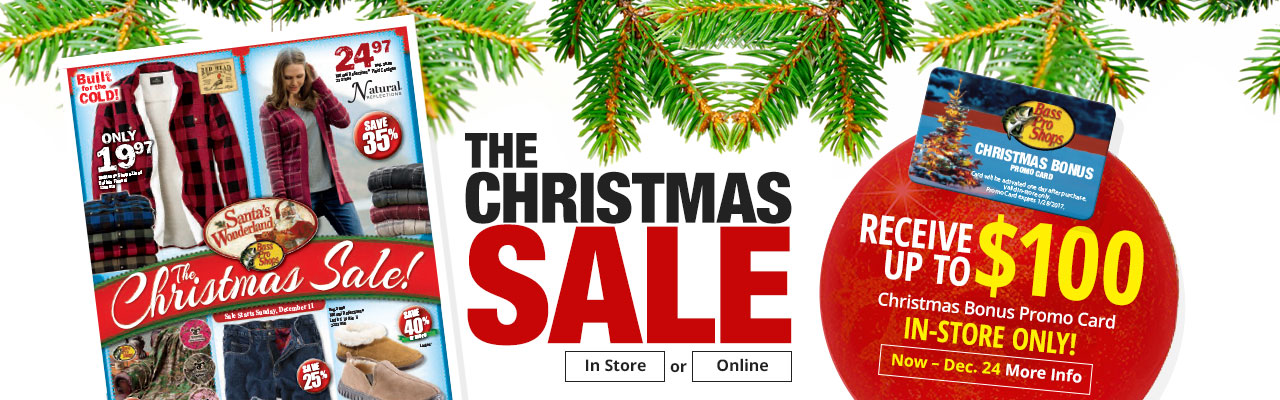The image depicts an online advertisement for Bass Pro Shop's "Santa's Wonderland" Christmas sale. The ad features holiday-themed visuals, including greenery from a tree at the bottom. To the left, there is a partial circular graphic with the text "Santa's Wonderland, The Christmas Sale."

At the top, the advertisement showcases a special offer on flannel shirts, declaring that they are lined and priced at only $19.97. The primary flannel shirt displayed is red and black, but the ad also shows a stack of additional color options, including blue, green, and an indiscernible shade. 

A section below highlights another offer featuring a woman wearing a similar lined shirt. This product is labeled as "natural," and is available for $24.97 after a 35% discount. A stack of these shirts in various colors is also depicted.

"Santa’s Wonderland” is visually featured in the center of the advertisement, with the text swooping in an arc. Beneath this, additional items are advertised, including lined jeans and fur-lined slippers.

A central banner in red pronounces "The Christmas Sale," with details indicating that the sale is available both in-store and online. The Bass Pro Shop logo is present, along with a promotion for a "Christmas Bonus Promo Card" offering up to $100 for in-store purchases made until December 24th. Clicking on the ad likely provides more information and options to shop online. 

The tagline humorously encourages shoppers with the phrase: "Go get your Bass Pro Shop stuff, because Santa does."